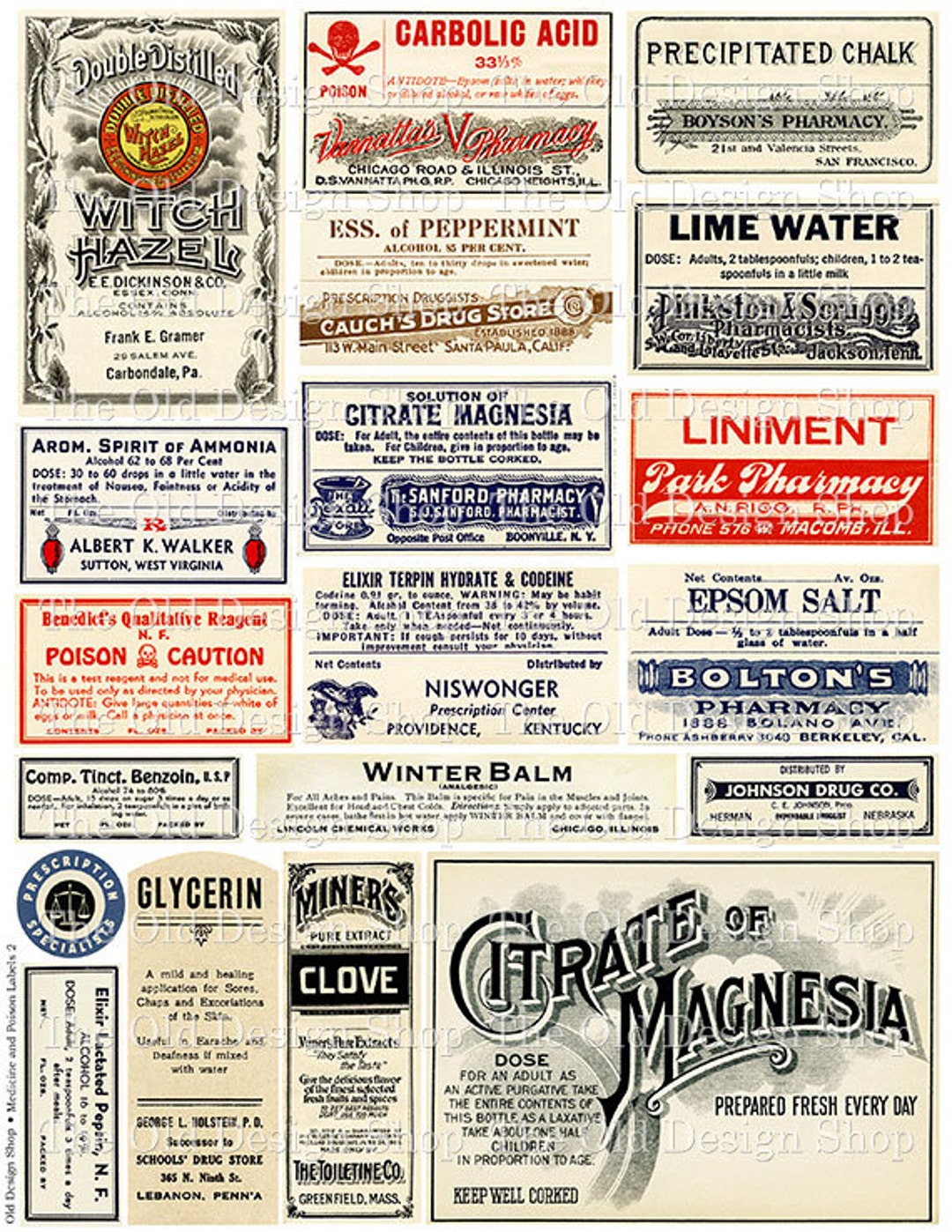The image appears to be a vintage page from the back of a local magazine, filled with a series of small, rectangular advertisements resembling business cards. There are approximately 12 to 15 ads, each promoting various medicinal and pharmaceutical products. The advertisements feature a diverse array of old-fashioned remedies and goods, such as "Double Distilled Witch Hazel" with a caution for poison, "Glycerin," "Miner's Clove," "Carbolic Acid," "Essence of Peppermint," "Citrine of Magnesium," "Winter Balm," "Precipitated Chalk," "Limewater," "Liniment," and "Epsom Salt." Some of the specific names and businesses mentioned include Epsom Salt at Bolton's Pharmacy and Liniment at Park Pharmacy. The ads collectively provide a nostalgic glimpse into the historical offerings of local pharmacies and medical suppliers.